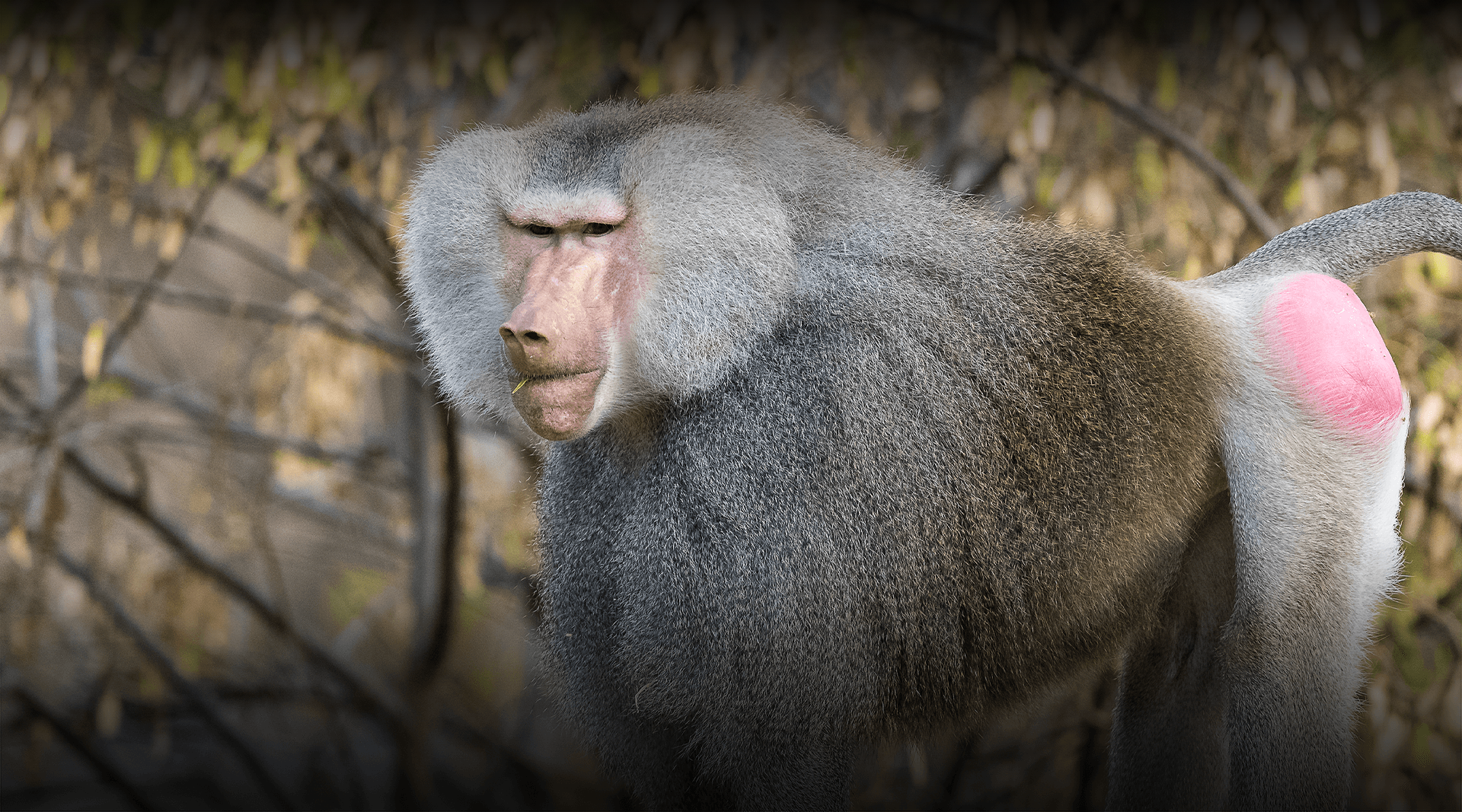The image is a detailed close-up photograph of a baboon, focusing on its unique and striking features. The baboon is standing on all fours in a forested area with an out-of-focus background filled with bare branches and some green leaves, providing a slightly hazy and vignetted ambiance. The baboon's fur is distinctly characterized by a mix of colors: grayish white fur around its head and shoulders, giving it a majestic, bushy look reminiscent of a lion's mane, and brown fur around its abdomen. Its rear hind legs are cloaked in light gray, white fur, contrasting with its bright pink, bare rump. The face of the baboon is flesh-toned with dark eyes and thick eyebrows that hang over its eyes, and its afro-like mane of fur spreads out from both sides of its face. It holds a piece of straw in its mouth, adding a touch of whimsical detail. The baboon's smooth tail extends out to the right, while it looks to the left, with its mouth close-set together, capturing a moment in nature with exquisite detail.